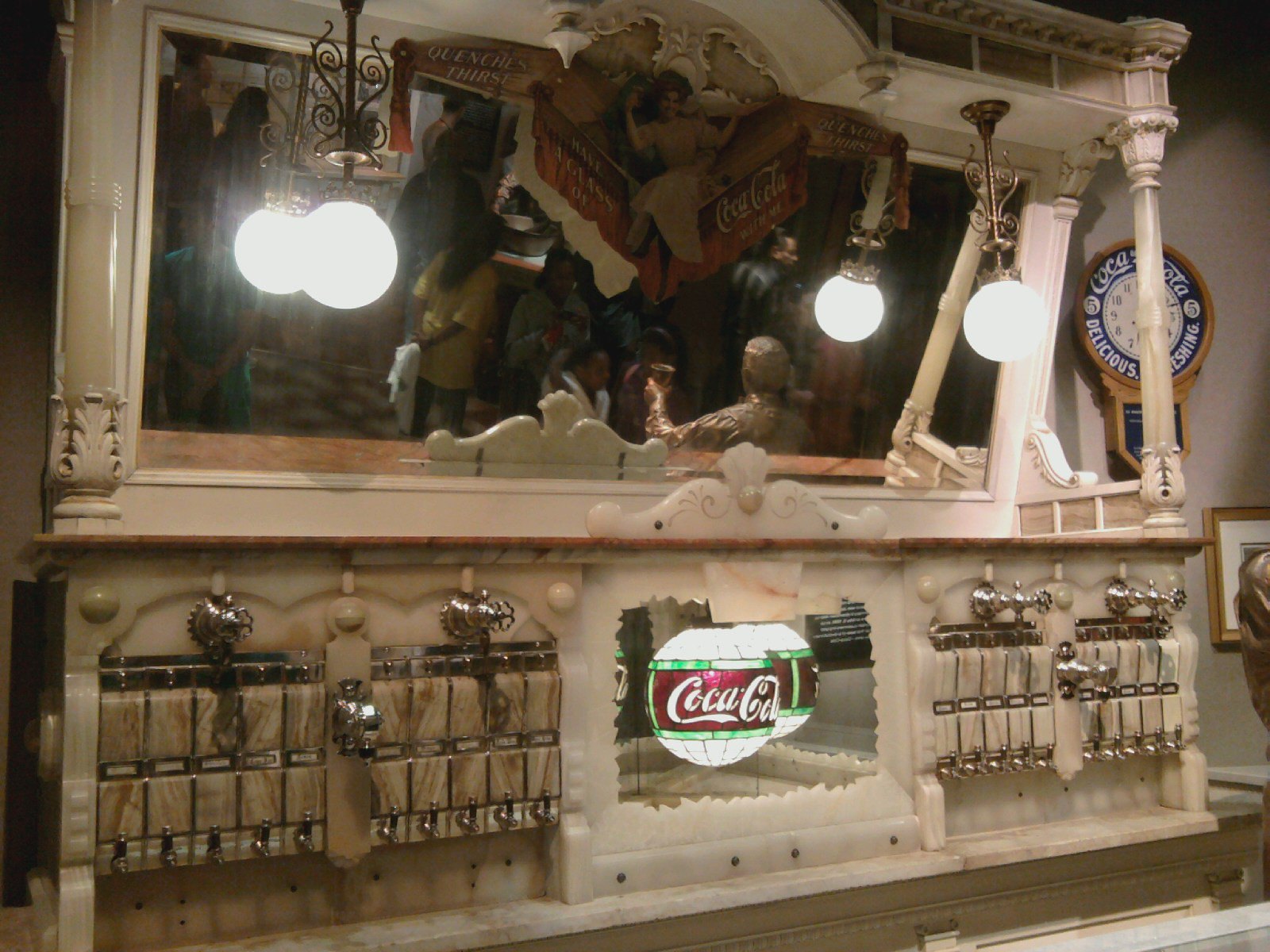This photograph, taken in landscape orientation, showcases a meticulously detailed vintage bar setup, possibly displayed in a museum setting. The bar is constructed primarily of wood painted in a delicate white or dark cream, featuring intricate leaf carvings on the side pillars. The bar is divided into two sections: an upper and a lower part. The top section features two hanging round lights and a large mirror, which reflects the bustling activity of people in the bar, adding depth to the scene. Below the main mirror, a smaller angled mirror enhances the vintage feel. Central to the lower section is a prominent stained glass Coca-Cola light, brightly lit and drawing attention. Flanked by spigots, potentially functional soda fountains or beer taps, this section adds an aura of authenticity to the bar setting. Additionally, a large clock with a white face and blue accents hangs on the wall, complementing the aesthetic. The overall scene is reminiscent of an old-timey soda shop or luxurious bar, capturing nostalgic elements in a refined wood finish that speaks to its high-quality craftsmanship.